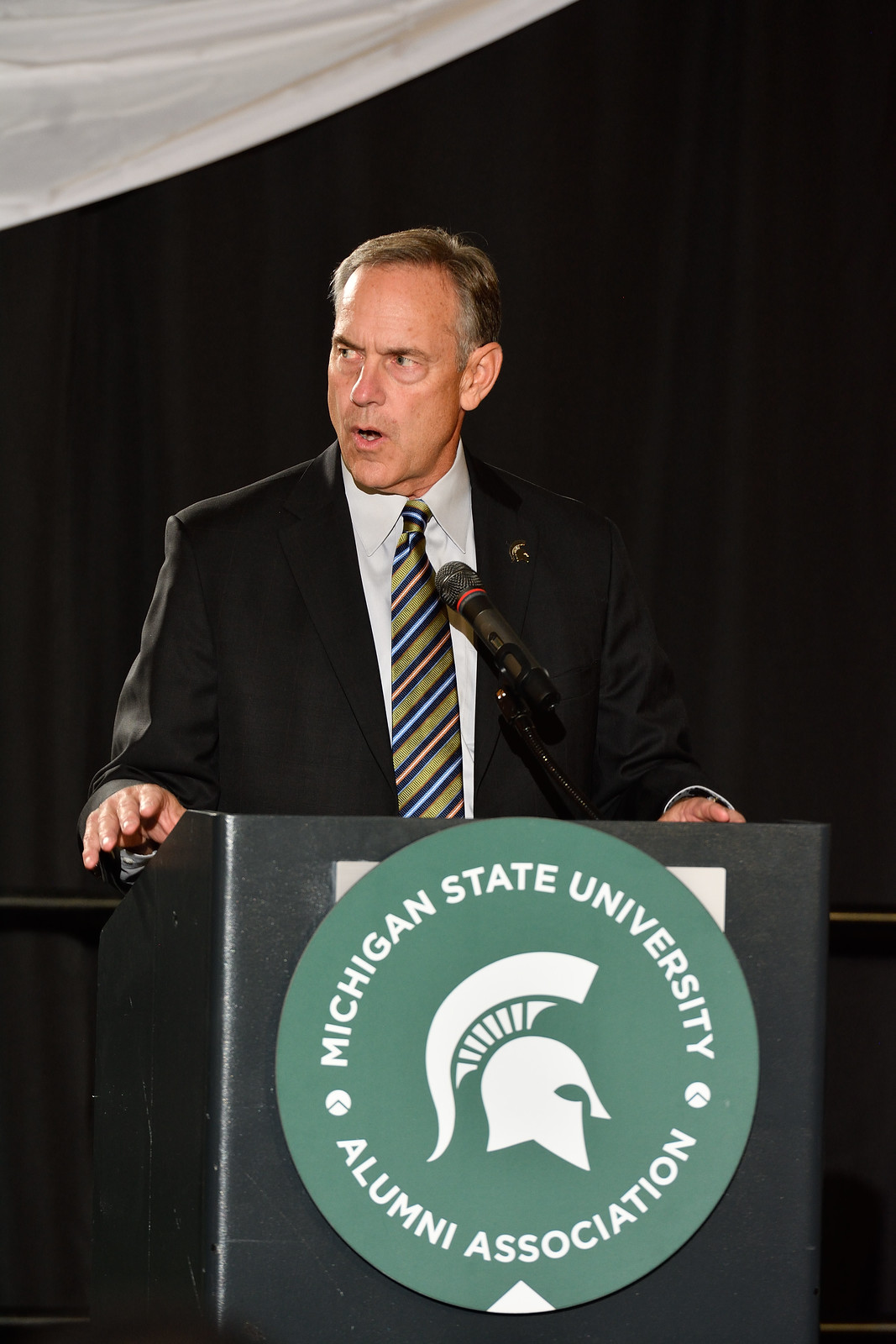In the image, a man is giving a speech at a Michigan State University Alumni Association event. He is standing centrally in front of a black podium, positioned behind a black and gray microphone on a black stand. The man has short brown hair, peach-colored skin, and is dressed in a black suit jacket over a white undershirt. His necktie features striped patterns in gold, dark blue, light blue, and light red. The school's circular logo, bearing white text on a green background, is prominently displayed on the podium. Positioned to the left of the logo is text that reads "Michigan State University Alumni Association." The man, captured with his mouth open and some teeth visible, appears to be speaking and is looking slightly to the left. The setting suggests a formal event, possibly a banquet, with a portion of a white curtain visible in the dark background, adding context to the scene.